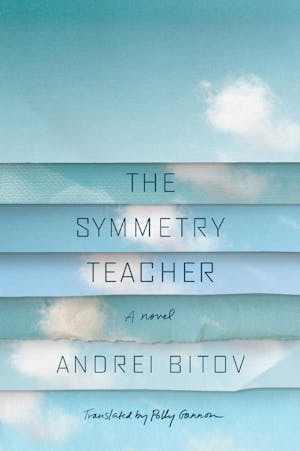The image is the front cover of the novel "The Symmetry Teacher" by Andrei Bitov, translated by Polly Gannon. The cover features an artful design of a blue sky with various shades, transitioning seamlessly, and dotted with clouds that sweep diagonally from the top right to the bottom left. This airy, serene background is segmented by lines into six uneven, overlapping sections resembling a stack of asymmetrical post-it notes or shutter strips, creating an impression of layered pages. The title "The Symmetry Teacher" and the author's name, Andrei Bitov, appear prominently, while the phrases "A Novel" and "Translated by Polly Gannon" are rendered in a lighter, script-like font, adding an elegant touch. The overall design is minimalist yet evocative, with a modern and slightly futuristic typeface, inviting readers into the contemplative and orderly world suggested by the title.